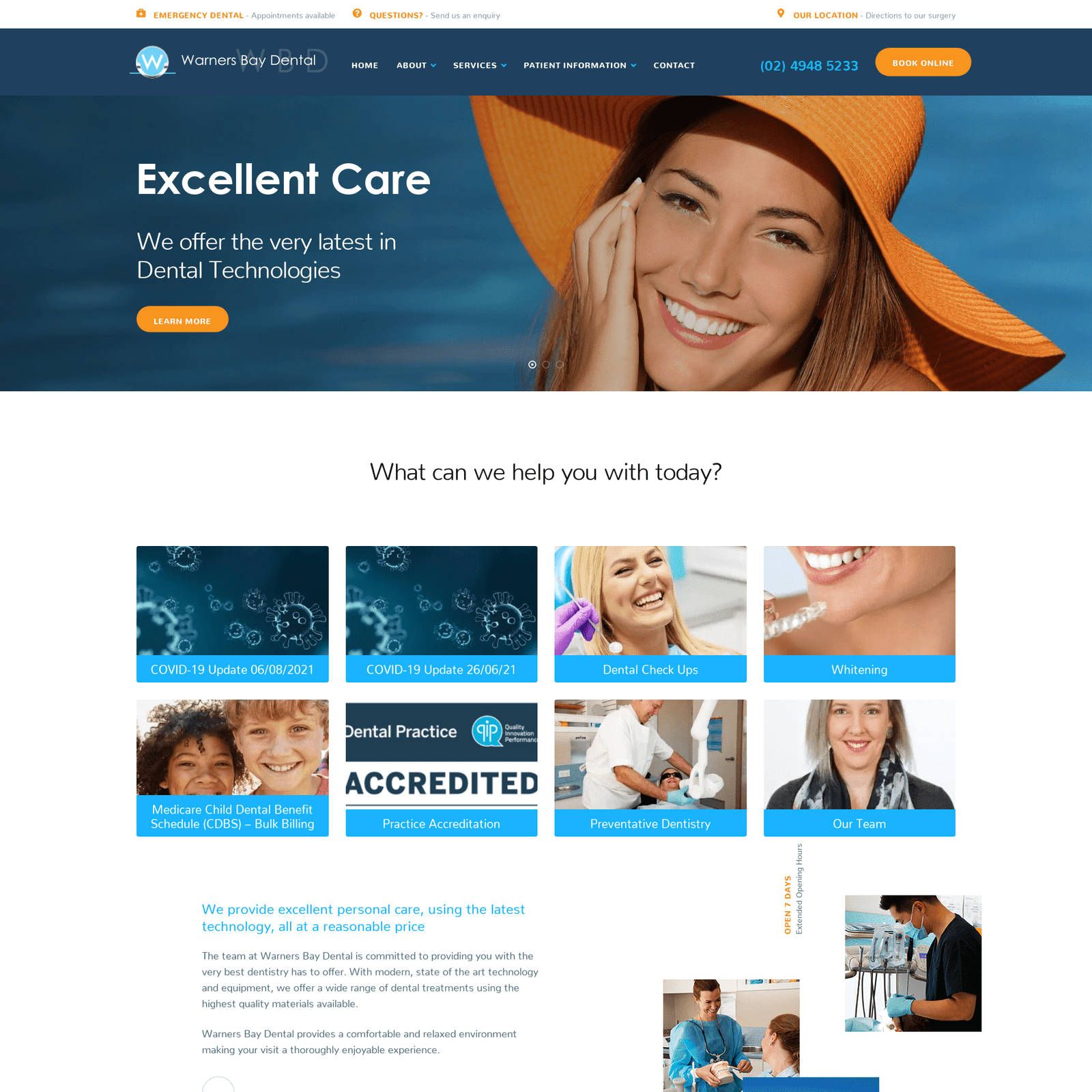The image depicts the homepage of the Warner Bay Dental website. The topmost section features a dark blue strip with white text displaying "Warner Bay Dental" on the left side, and the acronym "WBD" below it in a lighter font. To the right of this logo, the navigation menu includes options like "Home," "About" (with a dropdown menu), "Services" (with a dropdown menu), "Patient Information" (with a dropdown menu), and "Contact." Additionally, a phone number, 024-948-5233, is displayed next to an orange "Book Online" button on the right.

Above this blue section, there is a white background with orange and gray text that includes options for "Emergency Dental Appointment," "Questions," "Send Us an Inquiry," "Our Location," and "Directions to Our Surgery."

Dominating the middle of the page is a photograph of a smiling woman wearing a large orange floppy hat. She has a tanned complexion, brown hair, brown eyes, and is wearing a reddish-pink or peach-colored lipstick. The photo shows only her head and her right hand resting on her cheek. On the left side of the image, text in orange highlights the clinic's commitment: "Excellent care, we offer the very best in dental technologies." Below this text is an orange "Learn More" button.